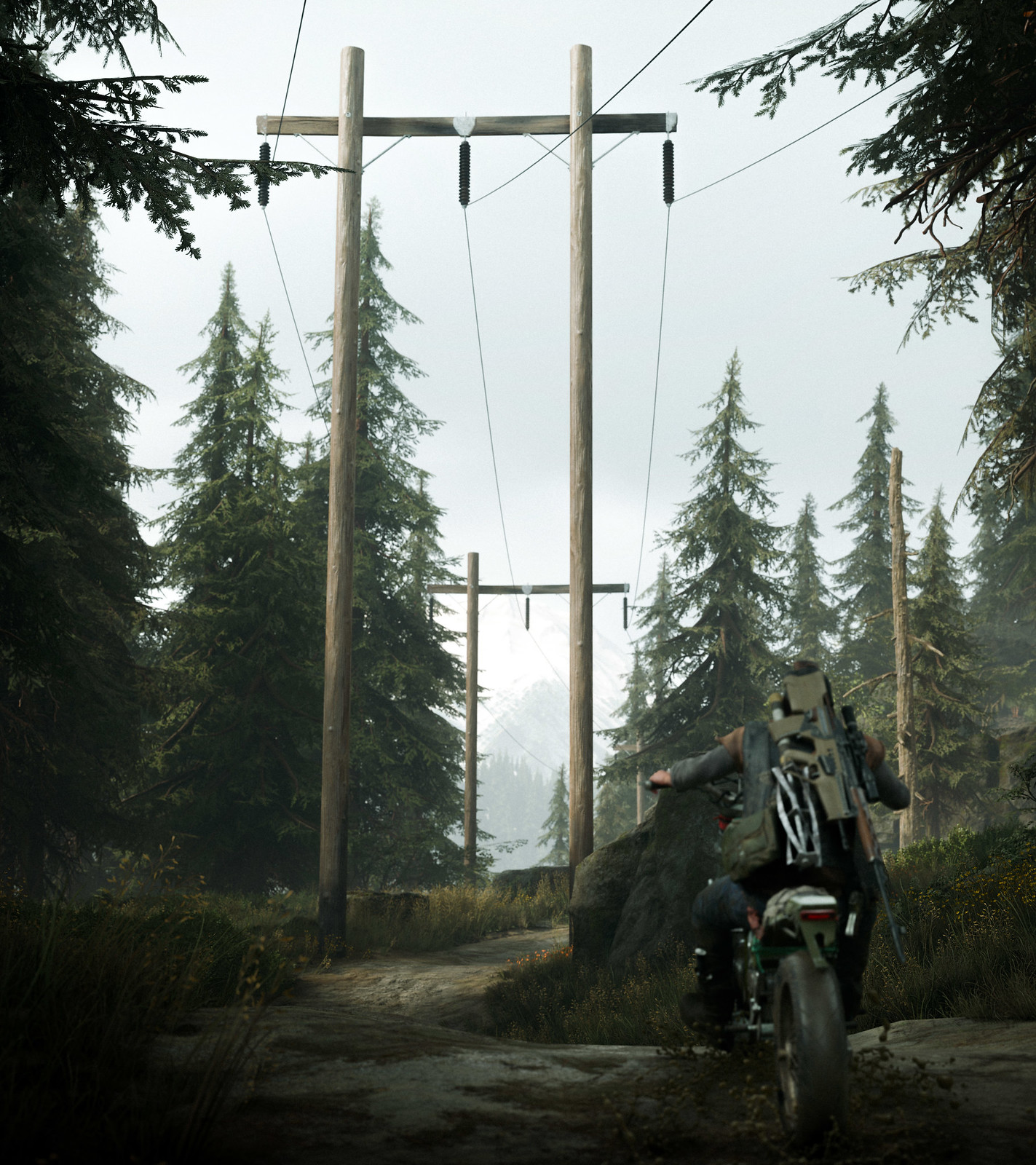In the image, a lone motorcyclist navigates a rough, unpaved dirt road through a sparsely wooded forest, characterized by tall fir and pine trees. He is dressed in long dark sleeves, a thick jacket, blue jeans, and a vest, riding a white or gray motorcycle with green accents, typical for rugged outdoor terrain. Strapped to his back is a large military-grade sniper rifle, suggesting a sense of preparedness for survival. An array of power lines, held up by wooden posts, runs parallel to the pathway, which is bordered by patches of tall grass, yellow wildflowers, and a large rock on the right. The sky overhead is a dull, whitish gray, adding to the somber atmosphere. The image, likely from a survival horror video game, hints at a narrative of isolation and endurance in a harsh, yet beautiful wilderness.